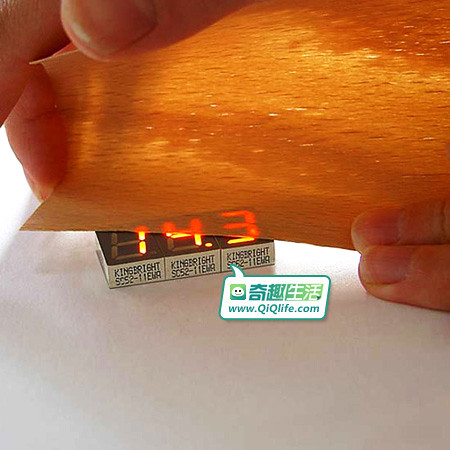The image appears to be a professionally shot photograph, likely intended for use in an advertisement. The setting features a pristine white table or surface, which hosts a sleek, rectangular electronic device. The device prominently displays the numeric value 14.3 in bright, hot orange-red digital digits. It’s divided into three sections, each beneath one of the digits, and labeled accordingly: the left section reads "King Bright 5552-11EMR," the center section is marked "King Bright SC52-11EMR," and the third section, partially obscured, also bears the "King Bright" label followed by "11EMR."

Two hands are carefully holding a transparent orange sheet over the top of the device, possibly suggesting an interaction or protective action. Adding an element of uniqueness and perhaps indicating the product's origin or brand, a small speech bubble emerges from the device. The bubble contains text in an Asian script, and below this writing, the URL "www.QIQLife.com" is clearly displayed, likely directing viewers to more information or the product's website.

This meticulously crafted scene, with its clean aesthetic and detailed presentation, underscores the modern, tech-savvy appeal of the electronic device, hinting at innovation and precision in its design and functionality.